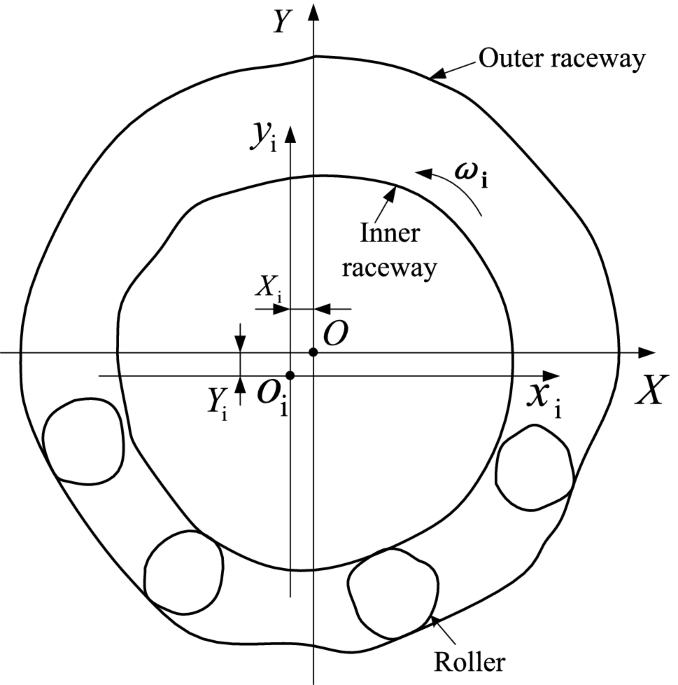The image is a hand-drawn graph depicting a combination of geometrical and labeled elements on a white background. The central feature of the graph includes a pair of concentric circles, with the inner circle labeled "inner raceway" and the outer circle labeled "outer raceway." These labels are indicated by black arrows pointing towards them. The graph has an X-axis extending horizontally to the right and a Y-axis extending vertically upwards, both clearly marked with capital letters "X" and "Y" respectively at their ends. Additionally, there are sub-axes labeled Y1 and X1. In the lower left and lower right quadrants of the graph, smaller hand-drawn circles are placed between the two main concentric circles, labeled "roller." Various rays and intersecting lines on the graph are labeled with subscript notations such as X_i, Y_i, and intersection points are marked with O_i, including the origin, which is simply labeled "O." This graph appears partly hand-drawn with some scribbly annotations indicating its informal nature.